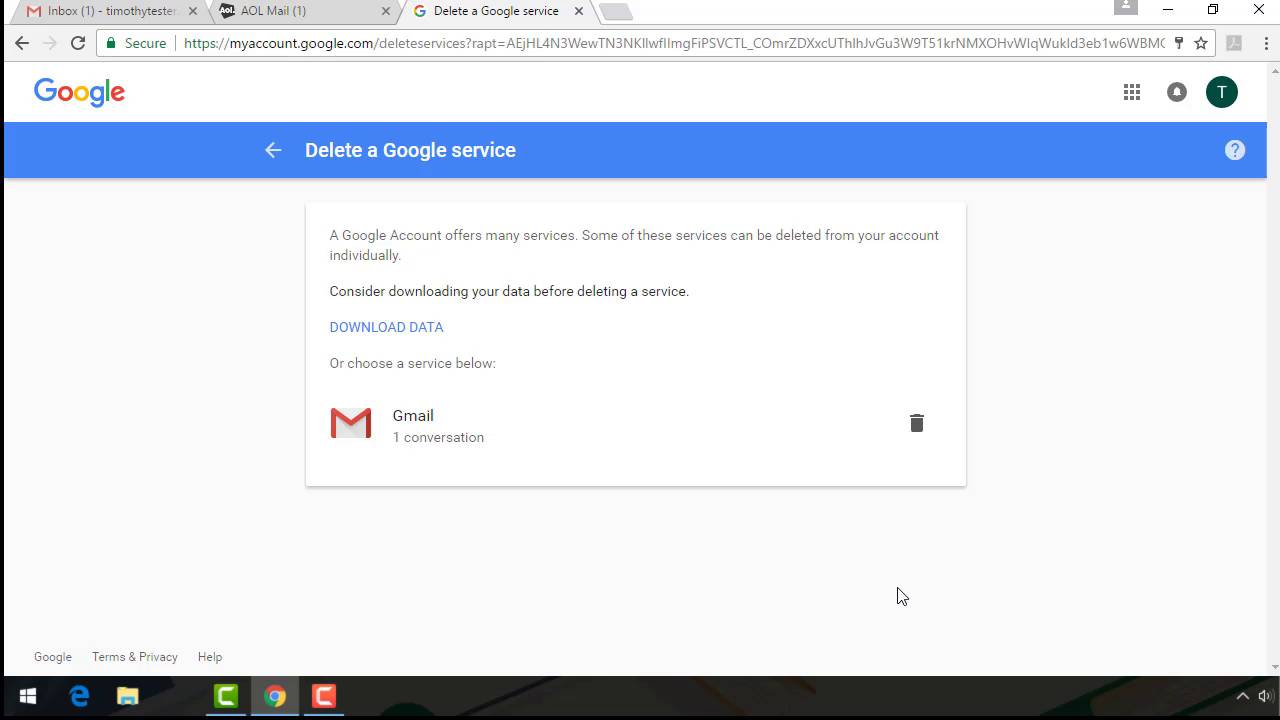The image depicts a web browser with three open tabs. The first tab is labeled "Gmail" and displays an inbox with one unread email under the name "Timothy Test." The second tab is titled "AOL Mail" and also shows one unread email with the name "Brinsey" next to it. The active tab is focused on "Delete a Google service," with the visible URL being myaccount.google.com. To the left of the web address are navigation controls: a back arrow, a forward arrow, and a refresh button. Below the navigation bar, the Google logo is visible alongside a profile icon, which is a green circle with a blue letter "T" inside. The main content area of this tab shows the "Delete a Google service" page, which includes a suggestion to download your data before deleting the service and a link to "Download data."